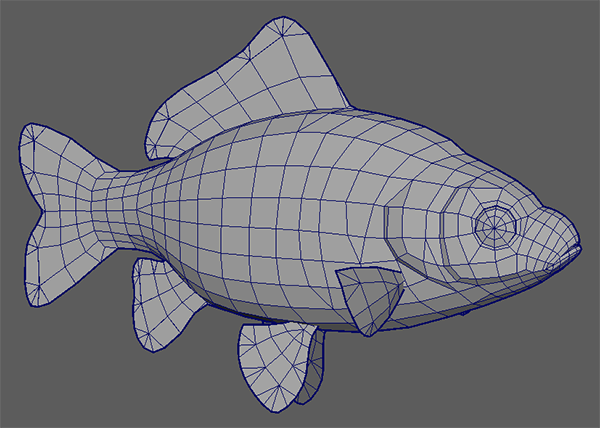The image depicts a digital 3D rendering of a fish set against a dark grey background. The fish is illustrated in light grey and brown hues, featuring a distinctly structured grid of dark blue lines that run across its body, creating a sense of depth and detail while possibly identifying various anatomical parts or scales. The head, eyes, and various fins are clearly defined, including a dorsal fin, two pectoral fins at the bottom, as well as another fin on the side and just behind the head. The tail fin is also prominently displayed. The overall setting and the color scheme emphasize the preparatory nature of this 3D model, showcasing the detailed planning involved in its creation.